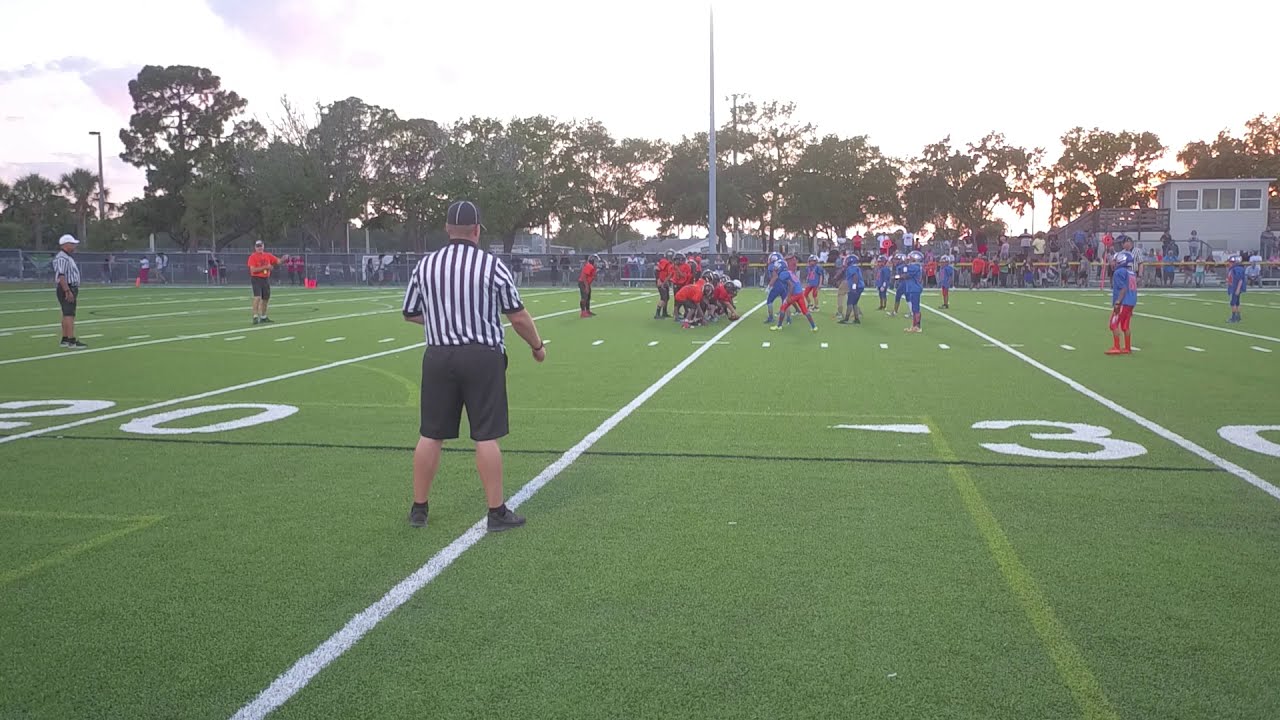This image captures a youth football game from a sideline vantage point on turf. The players, likely junior high kids, are lined up at the line of scrimmage on the 25-yard line, with the ball yet to be snapped. The team on the left is dressed in red jerseys with dark pants, while the team on the right wears predominantly blue jerseys with blue pants, with a few players donning red pants. A referee is prominently visible in the foreground, distinguishable by his vertical striped short-sleeve top, black shorts, and black and white cap. Another referee is seen on the left side of the field. The background features a crowd mingling near the trees under a sunny sky, indicating a late afternoon or early evening setting. Additionally, there is a fencing area with people standing both in front of and behind a barrier, and a temporary building is visible on the right-hand side of the image.